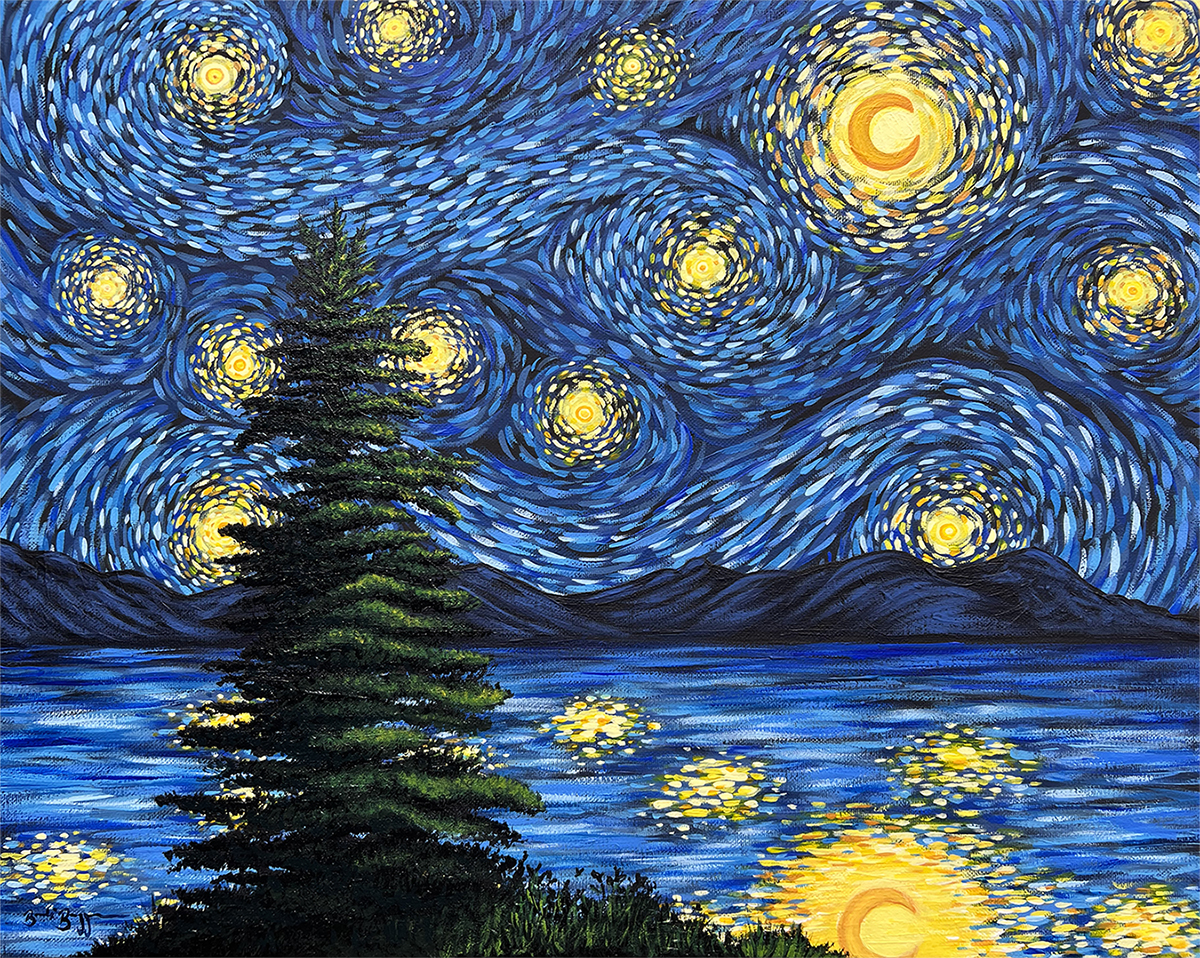This square painting is a detailed reimagining of Vincent van Gogh's "Starry Night," characterized by its mesmerizing swirled sky formed by dynamic patterns in varying shades of blue, interspersed with white dashes that create an impression of movement. Each swirling pattern harbors a sun or moon-like yellow circle, with a notable larger spiral in the upper right corner containing a crescent-shaped moon. The lower half of the painting features water reflecting the same yellow sunspots seen in the sky. Cutting across the middle of the painting are dark bluish-gray mountains stretching from left to right, providing a stark contrast to the vibrant sky. In the foreground towards the left side, an evergreen tree, reminiscent of a Christmas tree, stands tall against a grassy hill, replacing what was once depicted as a canyon and little houses in the original artwork. The tree is a new addition, diverging from van Gogh’s initial composition, and it adds a fresh element to this reinterpretation of the classic scene.